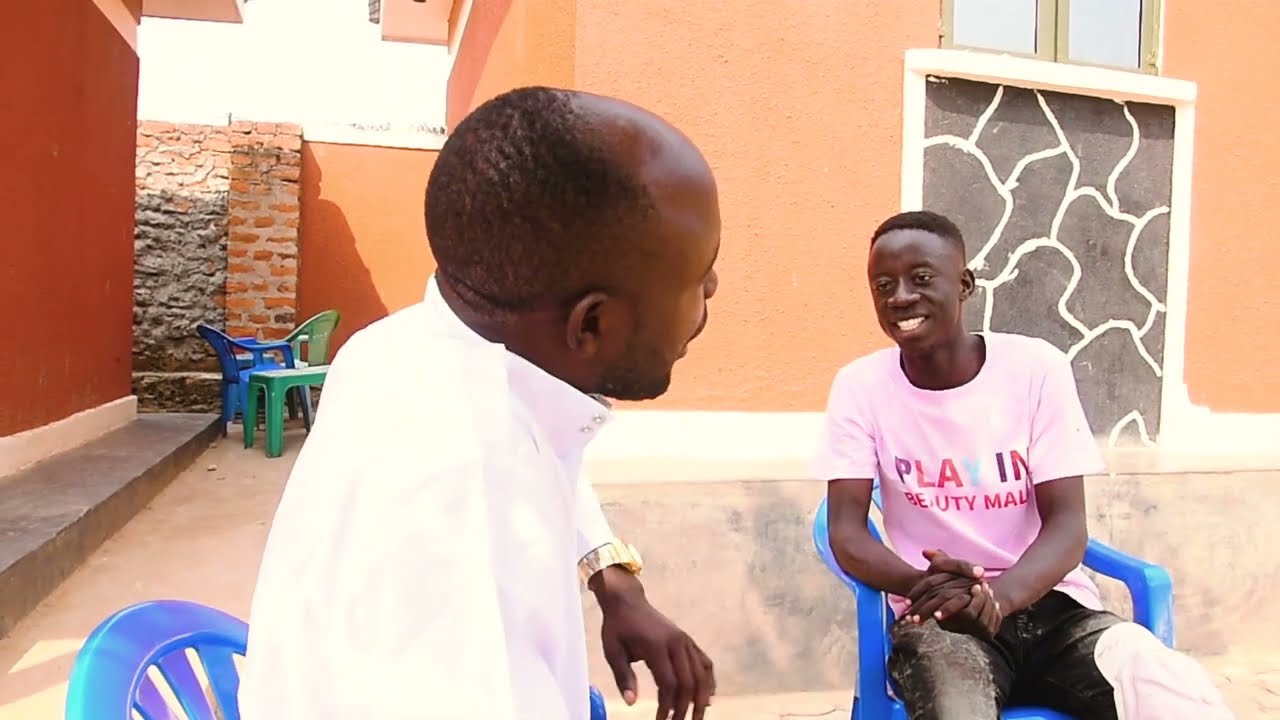In the image, we see two African-American men engaged in conversation outside in a residential area. They are sitting on blue plastic lawn chairs positioned on a creamy-colored walkway between two connected buildings, which are both orange with a mixture of stone and brick elements. The man in the foreground, wearing a white shirt and a gold wristwatch on his left hand, is seated with his back partially to the camera, revealing his half-bald head. He is looking to his right, speaking to the other man. The second man, directly facing the camera, is smiling broadly and wearing a short-sleeved pink t-shirt with the words "Play in Beauty Mall" in red, purple, and blue letters. He has short black hair and is dressed in black jeans. The scene is captured during the daytime, with the orange-colored buildings and a few scattered plastic lawn chairs visible in the background. Several windows can also be seen in one of the buildings.